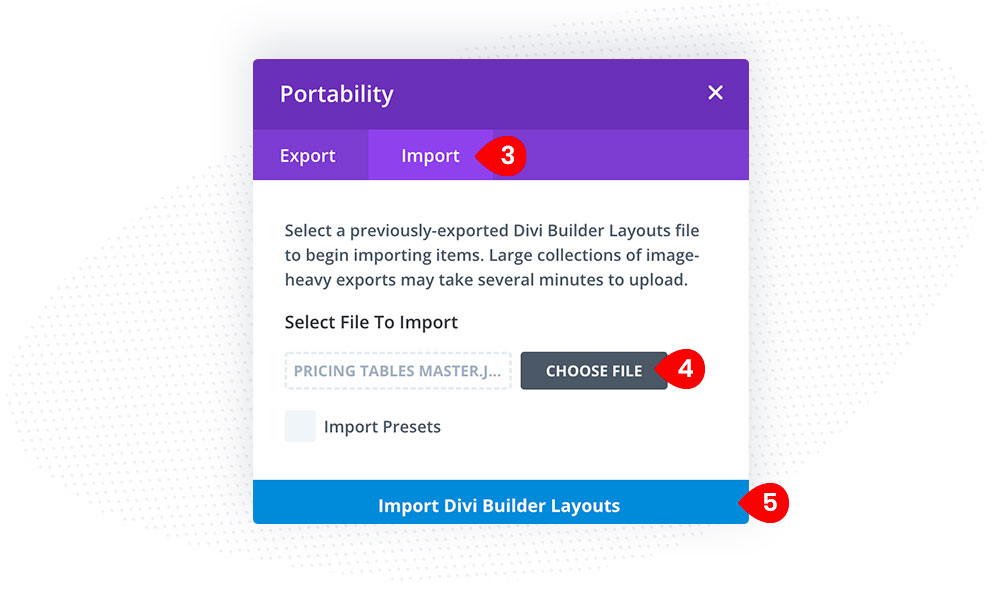The image features a user interface screen with a predominantly purple top section labeled "Tops." The screen provides daily access to various functionalities, including "purple export," "purple import," and "red pants."

Prominently displayed is a text message instructing users to "select a previously exported DB builder layout file to begin importing items," noting that "large collections of inventory exports may take several minutes to upload." The user selects a file to import, indicated by a message from an assistant, depicted as a dash marshmallow, which confirms that the "pricing table is mastered."

The screen also includes a grid labeled "juice file," displaying a setup that appears to have a sideways tar pick icon with the number four written inside of it in red. Below this icon is text stating "not choices," alongside options to "import presets" and "import DB builder layouts." Additionally, there is a sideways pin icon marked with the number five.

Behind the main window, there is a background grid pattern composed of numerous dotted lines. The overall background of the interface is white.

This detailed, descriptive caption captures the essence of the interface layout, specific instructions, and visual elements present in the image.